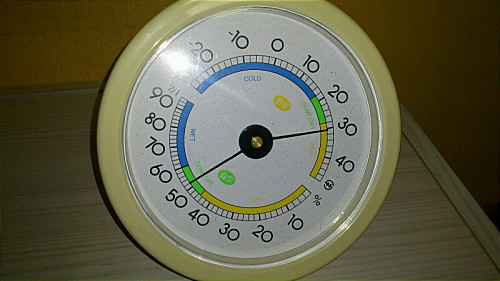The image features a wooden table, resembling Formica rather than real wood, set against a gold-colored wall. Atop the table sits a round, weather gauge instrument, reminiscent of a wall clock in shape but serving a different purpose. The gauge is meticulously detailed, displaying a range of numbers and percentages. 

Starting at the top, the numbers begin at zero and increment by tens in a clockwise direction: 10, 20, 30, and 40, each accompanied by the label "percentages." Following this, the scale continues on the right side from 10 to 90 in similar increments, looping back to the top. Additionally, from the top right position, negative numbers are also present: -10 and -20.

The gauge includes color codes: blue labeled "cold" and another segment in green, though the text is unreadable. The device also carries the labels "cold" and "wet," indicating it measures weather-related conditions such as humidity. Light shines on the gauge, highlighting its intricate details and making the colors and numbers more prominent.